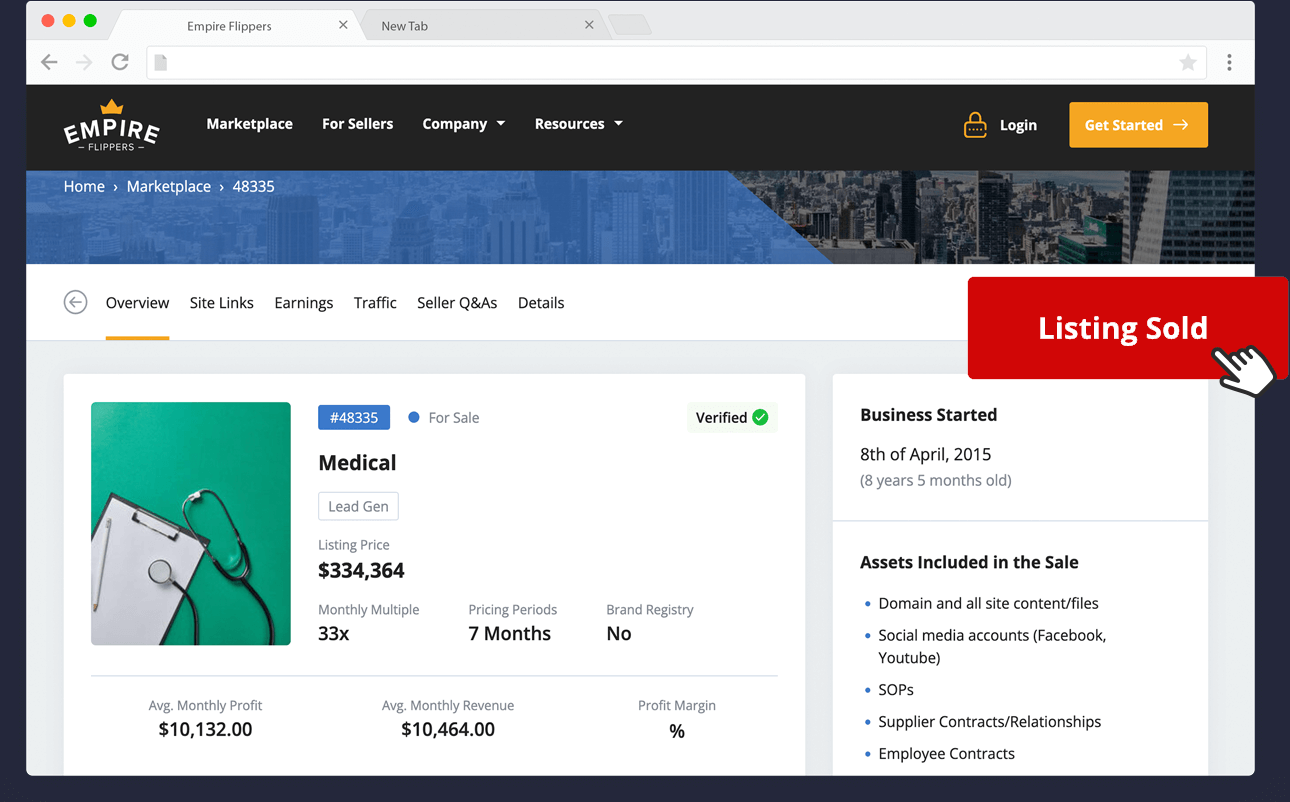"Empire Flippers: A Marketplace for Buying and Selling Website Domains

The website features a sophisticated design with intuitive navigation. At the top, there’s a sleek black border with white text for the main sections: 'Marketplace,' 'For Sellers,' 'Company,' and 'Resources,' with dropdown arrows indicating additional options. Below this, a blue border adorned with a cityscape image adds a dynamic, urban touch. 

Navigating further, the page prominently displays links to 'Home,' 'Marketplace,' and a specific product number, suggesting the website's focus on individual listings. The primary section of the webpage is predominantly white, bordered by subtle gray dividers that organize content seamlessly. Key terms like 'monthly multiple,' 'pricing periods,' 'brand registry,' 'listing price,' and 'for sale' are prominently featured in gray, highlighting essential information for prospective buyers and sellers.

To the right, a conspicuous red 'Listing Sold' button with white lettering is prominently displayed, accompanied by an icon indicating a hand or mouse click, symbolizing user interaction and emphasizing the website's commercial activity."